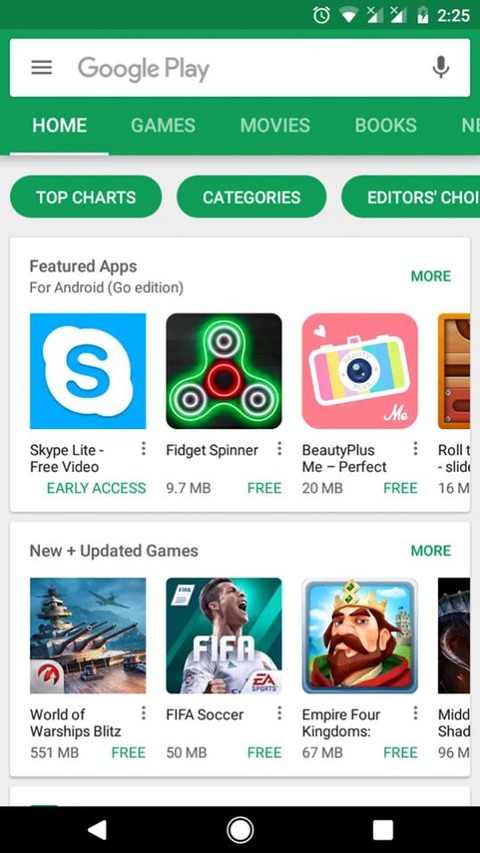This screenshot captures the Google Play Store interface on a mobile device. At the top right of the screen, the status bar displays several icons in sequence: an active alarm icon, Wi-Fi signal strength indicator, icons for SIM 1 and SIM 2 indicating no network connection, and a battery charging symbol. The device's current time, shown prominently in the corner, reads 2:25.

The main content of the screenshot features a selection of apps available on Google Play Store. The listed apps include 'Skype Lite,' 'Free Video,' 'Jet Spinner,' 'Beauty Plus,' 'World of Warships: Blitz,' 'FIFA Soccer,' and 'Empire: Four Kingdoms.' Each app is accompanied by its respective icon and likely includes some brief descriptions or ratings below each name. The overall image provides a snapshot of the user's current activity on the Google Play Store, offering insight into available app options and the device's status at the time of capture.